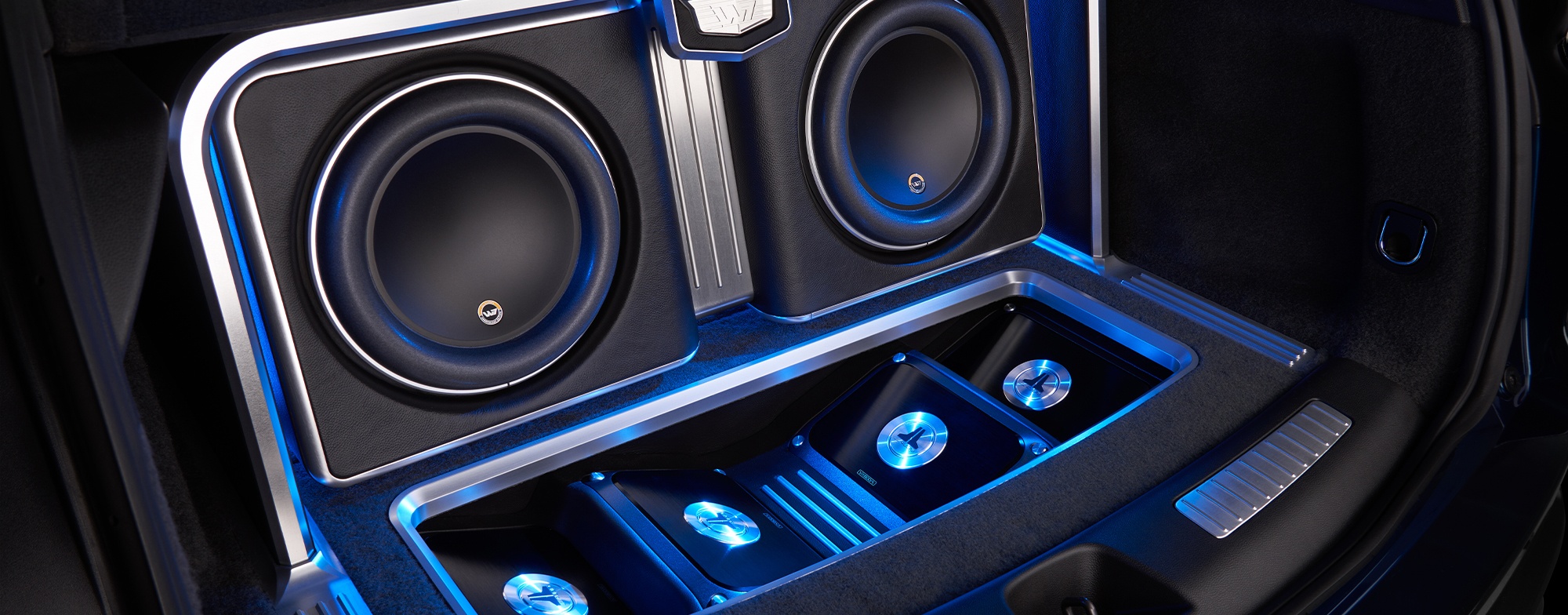The image depicts a close-up view inside the trunk of a dark blue car, focusing on a pair of built-in speakers. The main components visible are two black speakers, each adorned with an indistinct logo, possibly resembling a 'W'. These speakers are encased in a chrome or metallic frame, which adds a reflective quality that catches hints of blue light towards the bottom of the image. Below the speakers, the trunk features four smaller rectangular sections, primarily black with a chrome circle at their centers. The inner trunk environment is predominantly black, supplemented by silver accents, including a silver hook on the right and three silver strips on the otherwise black background. Black slanted sections flank the central area, each embedded with four silver circular areas, possibly indicating additional logos or functional elements. The detailed arrangement and metallic outlines suggest a high-end, custom audio setup within the car's trunk.